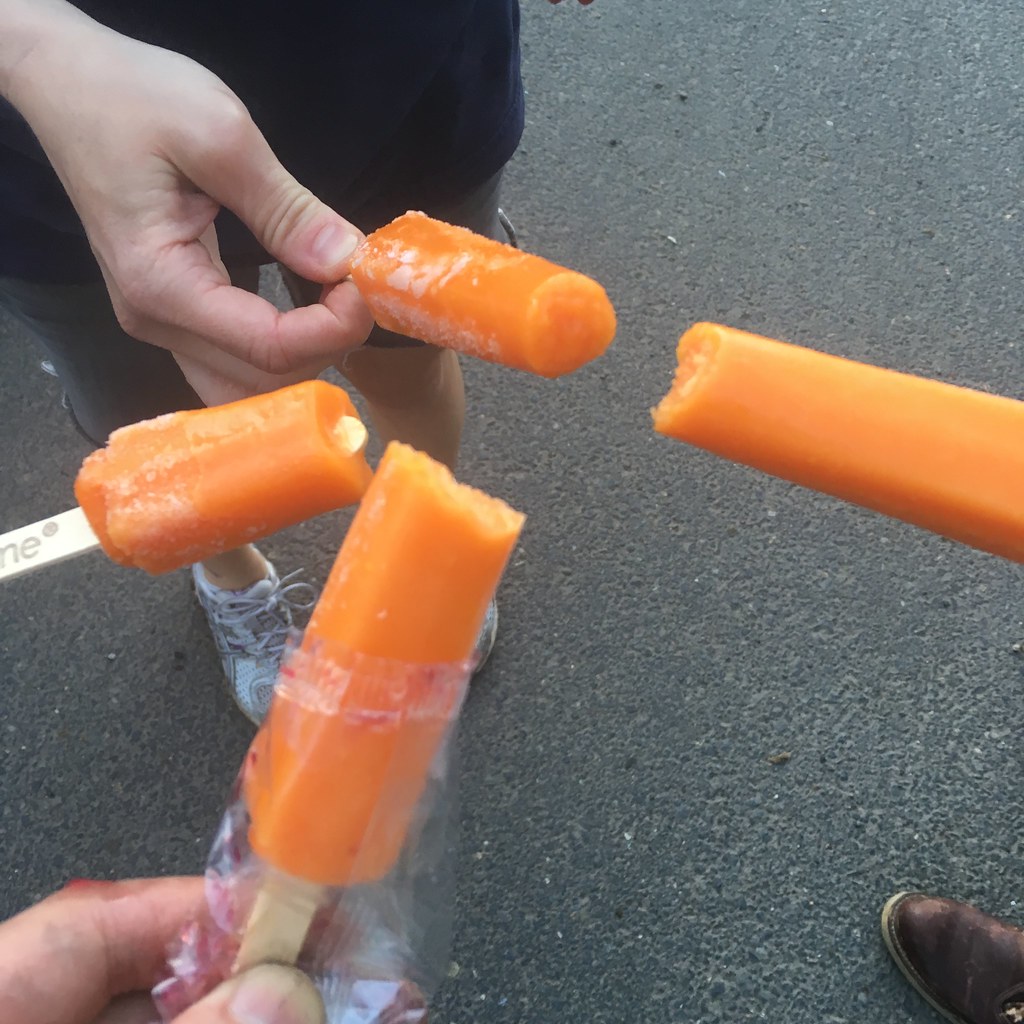In this square color snapshot, four partially-eaten orange ice lollies are held up in the air by what appear to be four different individuals, set against what looks like a parking lot or road surface. The image captures the lollies being showcased at varying stages of consumption, with the one on the far right eaten the least, and the one on the far left revealing the most of its wooden stick. The ice lollies are identical in type and are a bright orange color. 

In the upper left corner of the photo, a boy is visible, distinguished by his black shorts, black top, and trainers. His hand fully grasps the ice lolly. The lower left corner reveals a partial hand—showing just the index finger and thumb—along with the plastic wrapping around the ice lolly. The lower right corner shows a person wearing brown formal shoes, with only their ice lolly extending into the frame.

One of the sticks, in the middle, bears the text "NE" at the end along with a copyright symbol, adding a small, specific detail to the otherwise candid scene. The background features tarred wood, enhancing the informal and casual setting of the moment. The composition suggests a spontaneous photo taken to compare how much of their ice lollies each person has eaten.